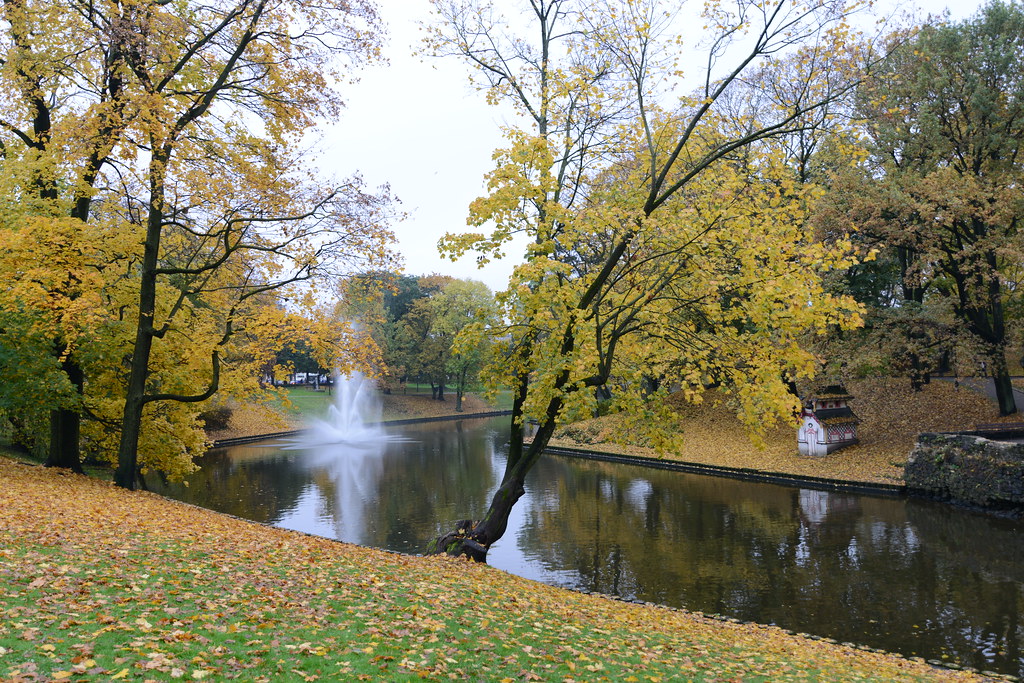This photograph captures a serene park scene in the fall, with a gently flowing stream or river curving into the background. The water feature includes a prominent geyser or fountain that sprays water approximately 20 feet into the air. The foreground features a lawn carpeted with yellow and brown leaves, while towering trees with matching autumnal foliage frame the scene on the left and center. Further back, more trees with vibrant yellow and orange leaves line the horizon. In the middle right background, a quaint, Japanese-style hut with a white facade and black slats on its pointed roof adds a charming architectural element. The banks of the water are well-constructed and lined with concrete, enhancing the idyllic and orderly appearance of this tranquil fall landscape. The sky is a bright white, contributing to the overall luminance of the scene, and there are no people or animals in sight, emphasizing the peaceful solitude of the moment.